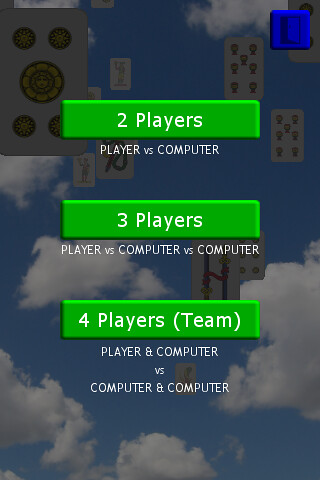The image is a vibrant, color screenshot from a video game or app screen. The backdrop features a partly cloudy blue sky with floating rectangular card-like images or dominoes drifting amidst the clouds. In the top right corner, there is a deep blue button with an icon resembling a partially open door, likely functioning as an exit button. Centrally located are three bright green buttons aligned vertically, each with white text detailing different gameplay modes. The top button reads "Two players," with "Player versus computer" underneath. The middle button states "Three players," followed by "Player versus computer versus computer." The bottom button indicates "Four players (team)," with the description "Player and computer versus computer and computer."